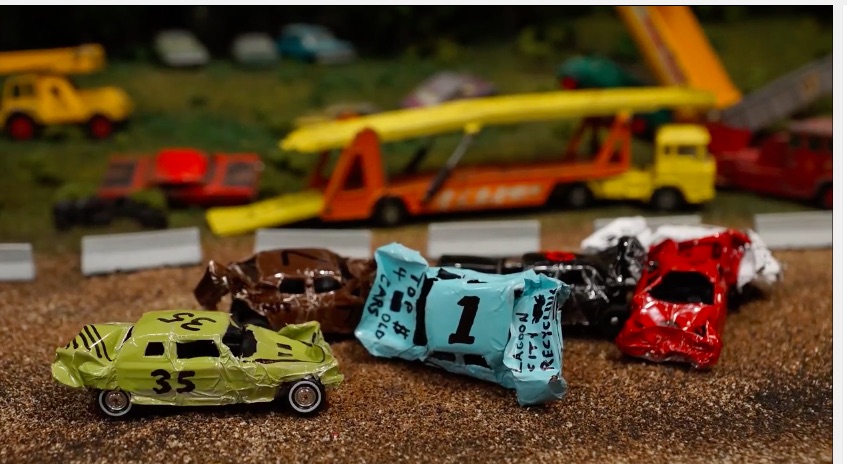The photograph features a meticulously crafted diorama that simulates a crash at a racing event using miniature die-cast cars, likely resembling Hot Wheels or Matchbox models. The forefront of the image showcases several vividly detailed cars with visible damage, likely custom-made or altered with tools to appear crumpled and weathered. Most prominent among them is an olive-colored car marked with the number 35, featuring striped details and extensive crash damage. Nearby lies a light blue car, flipped on its side and severely crushed, emblazoned with the number 1 and bearing the slogans "Top Dollar for Old Cars" on the hood and "Lagoon City Recycling" on the back, suggesting the scene might double as an advertisement mock-up.

The scene also includes a brown car with the number 7, a red car, and a black car, all of which are similarly battered. These vehicles rest on a gravel road, surrounded by detailed replica barriers, akin to those used in actual racing events to control traffic. Adding to the realism, a large orange and white car carrier truck is positioned behind the primary wreckage, with more out-of-focus vehicles and a grassy setting visible in the hazy background. The distant backdrop is rendered as pitch black, emphasizing the chaotic, wreckage-heavy foreground. This scene is reminiscent of a child's play set that's been intricately styled to resemble a junkyard or a dramatic racing crash site.